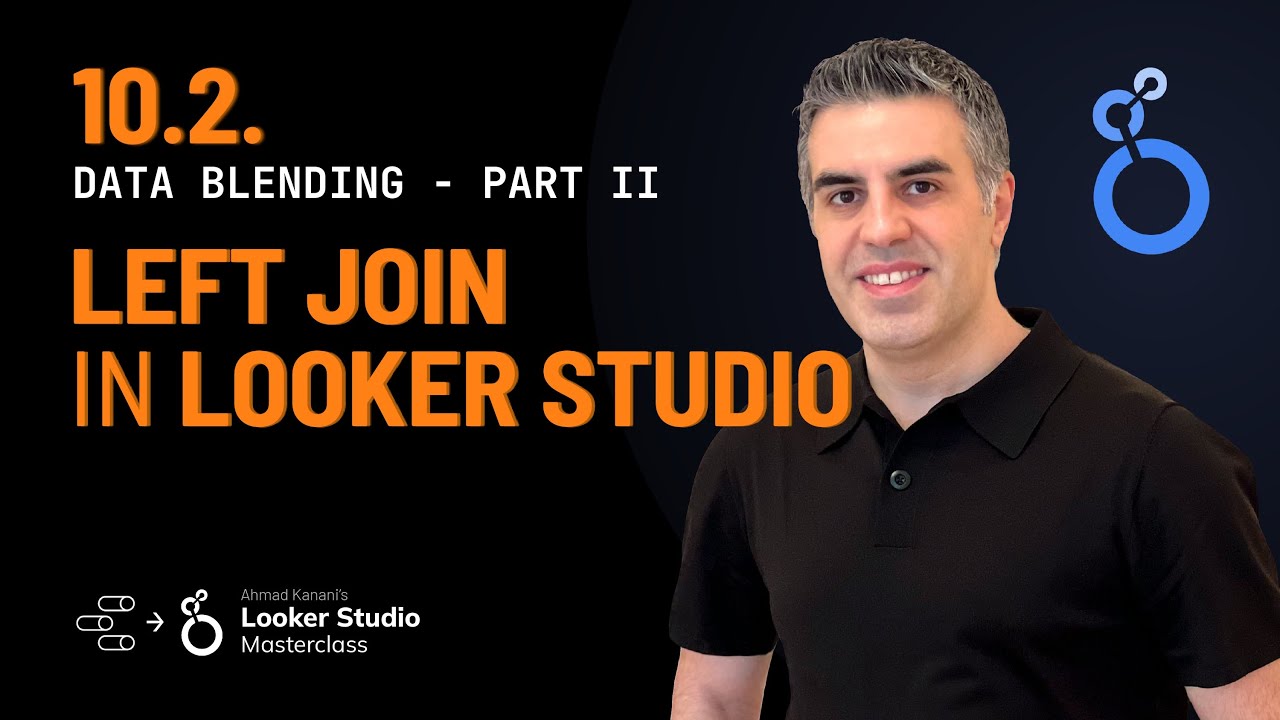A detailed descriptive caption could be:

"This screenshot from a website features a well-designed layout with both visual and text elements. On the right side, a light-skinned man with slicked back, mixed gray and black hair smiles at the camera. He is dressed in a short-sleeved, button-up shirt with a neatly pressed collar. Adjacent to him is a dynamic blue circular graphic: a set of concentric circles in varying shades of blue, interspersed by a black line that disrupts the outermost ring. On the left-hand side, an orange label displays '10.2,' followed by the white text 'Data Blending - Part II,' where 'II' is in Roman numerals. Below this, in orange, it says 'Left Join in Looker Studio,' with 'Looker' spelled out as 'L-O-O-K-E-R.' Positioned on the lower left are three pill-shaped sliders, arranged in a cascading manner with an arrow pointing from them to the blue circular graphic. Below this arrangement, in gray text, the name 'Ahmed Khanis' is displayed, followed by a bold white 'Looker Studio Master Class.' This composition effectively combines visual appeal with informative text."